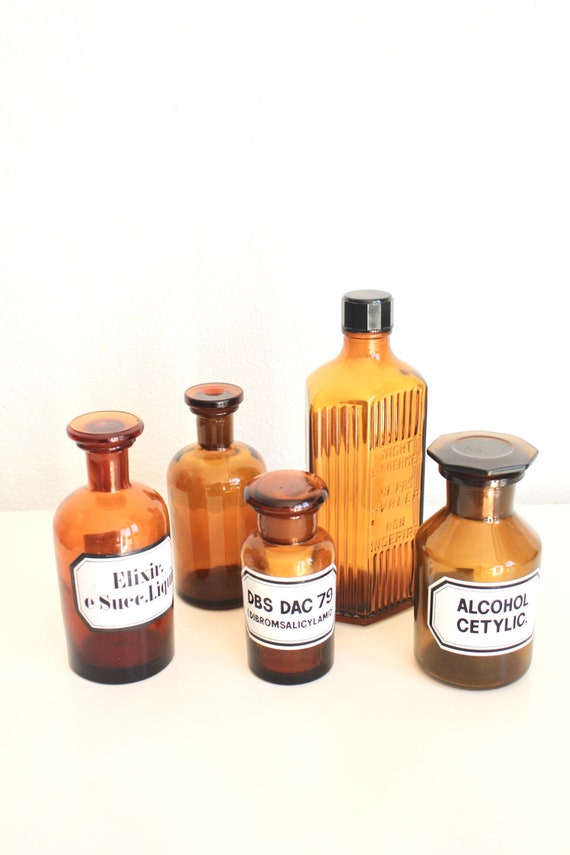This image showcases a set of five vintage-style amber glass bottles, placed on an off-white ground against a plain white background. The bottles vary in shape and size, with most featuring glass stopper tops, except for a taller, ridged bottle with a black screw top. This particular bottle, shaped like a rectangle, appears more modern compared to the others. At the forefront, three round bottles of different sizes dominate the scene with distinct black and white labels. The leftmost bottle's label reads "elixir" followed by an illegible word and then "liquid." The smallest bottle in the center displays "DBS DAC-79" along with some unreadable smaller text. The furthest right bottle has "alcohol" prominently labeled, followed by the partially legible word "cetyl." Two other bottles, one of which is blank and possibly empty, complete the set. Despite their vintage appearance, the bottles are impeccably clean and well-maintained, suggesting they might be replicas designed to look old.